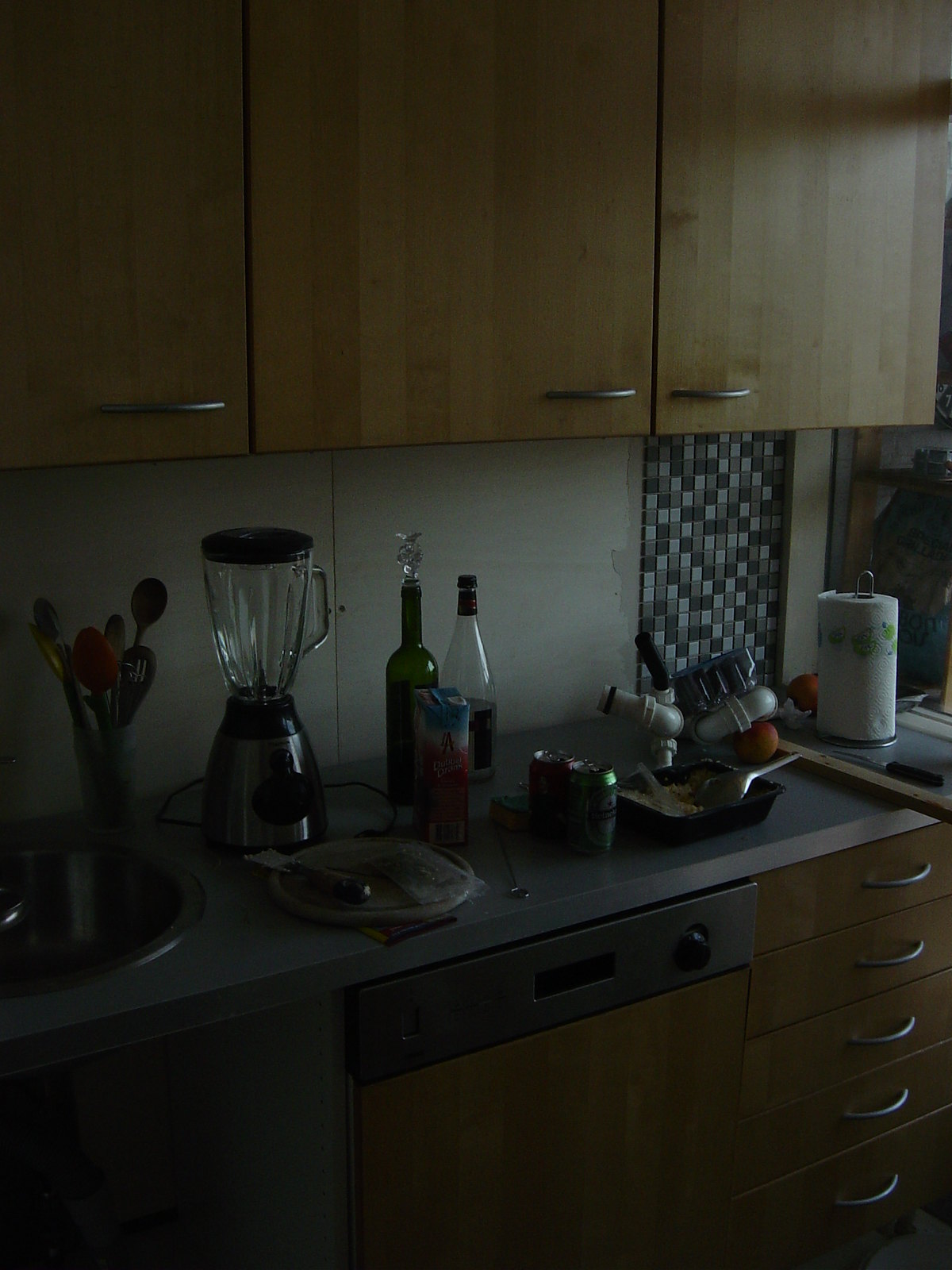This image captures a slightly dim kitchen illuminated by a light source coming from the right, possibly through a window. The cabinetry, both upper and lower, is made of a light brown wood, each adorned with sleek silver handles. The countertop below is a gray color, hosting a variety of kitchen items. 

On the left side of the kitchen, there's a metal sink integrated into the gray countertop. To the right of the sink, a silver dishwasher is visible, featuring a black handle and a matching black control panel. The countertop also holds a utensil holder filled with ladles, a stylish blender with a silver base, a black handle, and a glass pitcher. Below the blender, a circular object sits, though it's not clearly identifiable.

Next to the blender is a green bottle, a clear bottle, and a plastic container. Two cans are placed near these items. To the right of these cans, there is a black utensil holder containing a metal fork. Beyond this, there are some oranges, white kitchen gadgets, and a roll of paper towels.